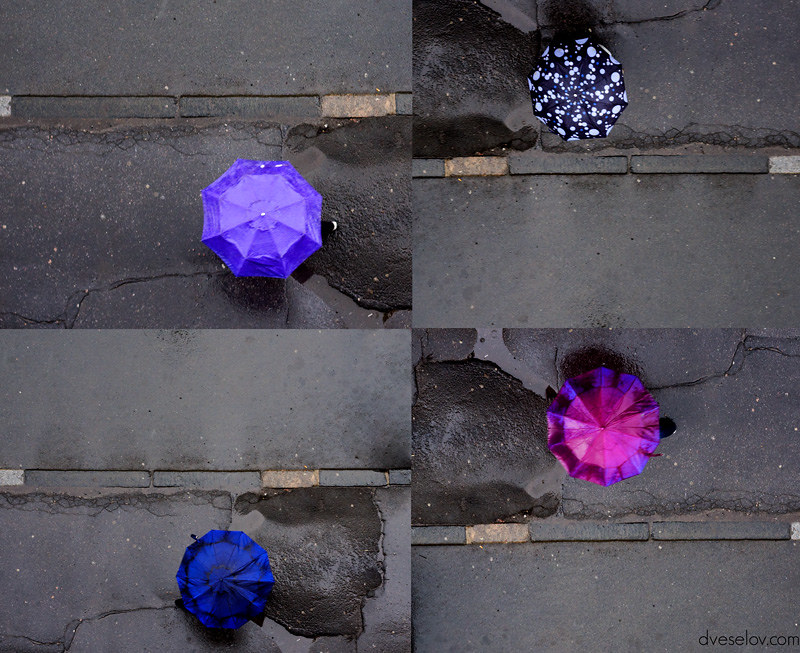An aerial photograph consists of four quadrants, each showcasing a different umbrella against a background of asphalt and sidewalk, which features various markings. In the top left quadrant, a dark blue umbrella with black trim is positioned next to a small puddle on black asphalt marked with faint orange stripes. The top right quadrant displays a striking black umbrella adorned with white specks of varying shapes and sizes, bordered by a yellow marking and overshadowed by a curb. The lower right quadrant features a vibrant pink umbrella with a burgundy trim around the edge, positioned above a mix of blue and purple hues. Finally, the lower left quadrant frames a light purple umbrella with a matching trim next to a puddle, set against asphalt with subtle curves and lines. Each segment captures the umbrellas from a slightly shifted vantage point, providing a comprehensive and varied depiction of the scene below.